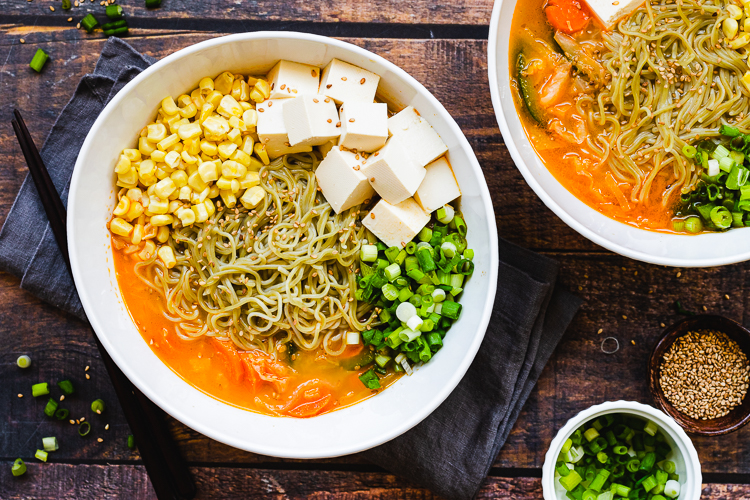This overhead photograph captures a mouth-watering display of food set on a rustic, slatted wooden table that resembles a picnic setting. The main focus is a white porcelain bowl filled with thin yellow noodles at the center, meticulously arranged with multiple ingredients segmented around it: corn kernels on the upper left, cubed tofu on the upper right, topped with toasted sesame seeds, and finely chopped green onions on the lower left. A reddish broth or sauce fills the remaining section, adding a vibrant touch to the composition.

Accompanying the main bowl are additional elements on the table: a small white bowl contains more chopped chives, and a brown bowl holds extra sesame seeds. Adjacent to these, black chopsticks rest on the left of the main bowl. Another white porcelain bowl, slightly smaller yet similar in size and adorned with an identical mix of ingredients, is positioned in the upper right corner. Interestingly, this second bowl also boasts bright orange elements, likely squash, completing the visual feast. Scattered chives on the table and the neatly folded cloth napkin under the main bowl add an extra layer of detail and texture to this beautifully arranged culinary scene.